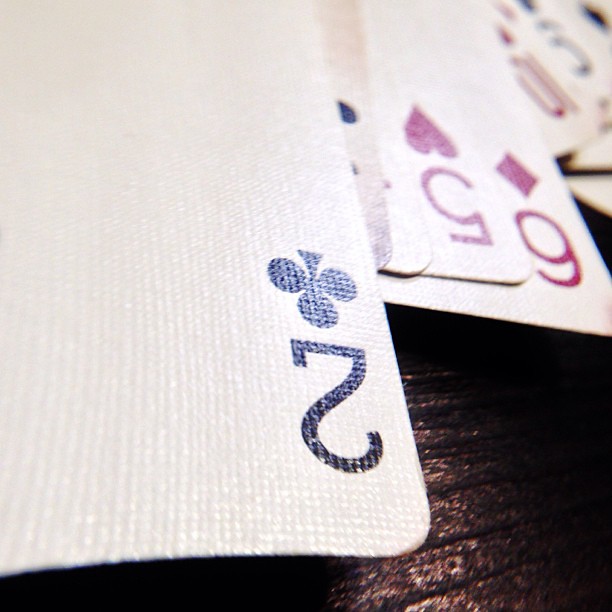A close-up shot of a deck of cards spread out on a table. The two of clubs, positioned upside down, takes center stage in crisp focus. Behind it, only partially visible, are the five of hearts, six of diamonds, a red ten, and a black nine, their details progressively blurring as they recede into the background. The image captures the intricate textures of the cards, revealing their individual fibers and ridges arranged in a perpendicular grid. The deck rests on a black table, possibly made of dark wood, hinted at by an occasional streak of green in the background.